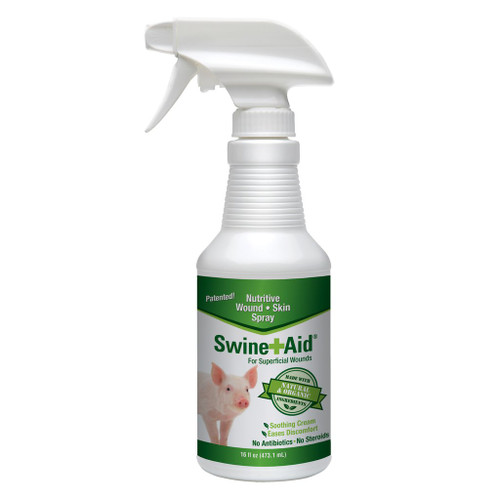The image features a centrally positioned, white spray bottle set against an entirely white background, giving it a clean, product-focused appearance ideal for a sales website. This opaque bottle is adorned with a green and white label and has a trigger spray mechanism. The top and bottom sections of the label are green, sandwiching a white middle section. The prominent text on the green sections includes "Patented Nutritive Wound Skin Spray" at the top and additional details at the bottom, though partially unreadable. The central white section reads "Swine Aid" in large green letters, followed by "for superficial wounds." A green ribbon beneath highlights "natural and organic," with nearby small circular seal affirming the same. A pink pig icon appears on the left side, adding a visual cue related to the product's intended use. Further down, it notes "Soothing Cream, eases discomfort," and assures "no antibiotics, no steroids." The bottle holds 16 fluid ounces of product.